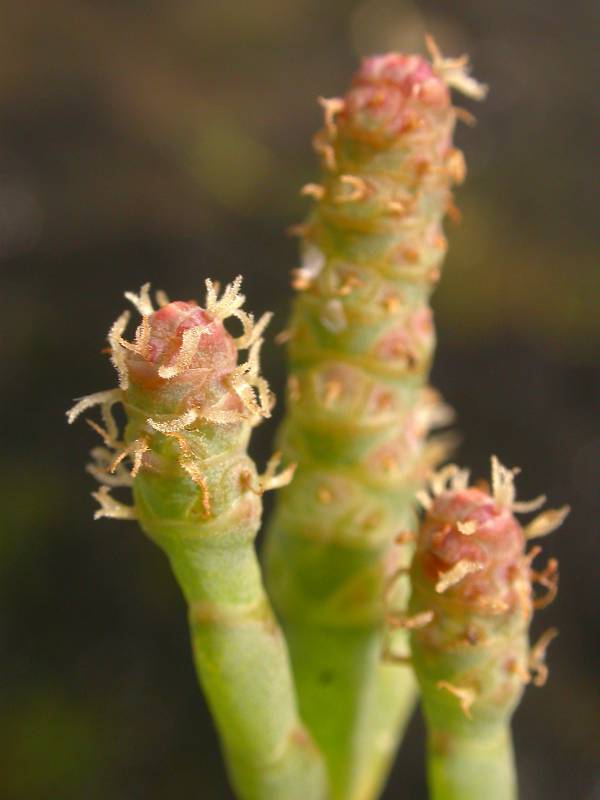This close-up photograph captures a detailed view of a plant's bud in a natural outdoor setting. The main focus is on three cylindrical, bird-like buds emerging from the plant. These buds have a green base that transitions to a vibrant red at the tip, accented by light brown and golden strands or fibers extending from them. The two smaller buds at the front are tall and slender, while the thicker bud in the background bulges near its middle and features scattered pink hues intermingled with the spiky fibers. The blurred background showcases various shades of green and black, indicating a surrounding of other plants and possibly trees, adding depth to the image without detracting from the focal buds. The photo is taken in portrait orientation under bright, natural light, effectively highlighting the intricate details of the plant.